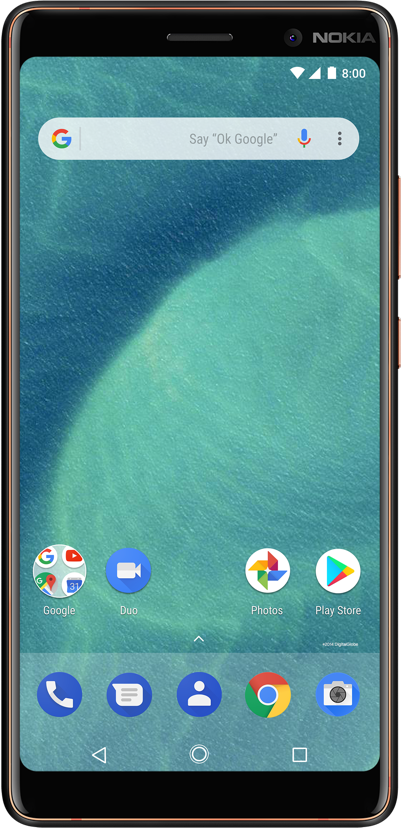This photograph showcases a sleek black Nokia smartphone set against a pristine white background. Prominently displayed on the top right corner of the phone is the "Nokia" branding, adjacent to the camera and speakers. The phone's screen background features a serene water image in shades of blue and green.

At the very top of the screen, a Google search bar is visible with the text prompting, "Say OK Google," accompanied by a microphone icon and three dots. Below the search bar lies an array of essential applications. The first app is a Google folder, depicted as a circular icon containing shortcuts to several Google services like Calendar, Maps, YouTube, and Google Search. Following this is the Duo app, represented by a webcam icon; then the Photos app, which has a colorful pinwheel design in blue, green, red, and yellow. The Play Store app is next, easily recognizable by its white circular icon featuring a multicolored Play logo.

At the bottom of the screen, the essential apps section includes: the Call app, Message app, and Contacts app, all depicted in blue with white icons; followed by the Chrome browser and the Camera app. Finally, at the very bottom, the navigation keys consist of a Back button, a Home button, and a Square button for recent apps.